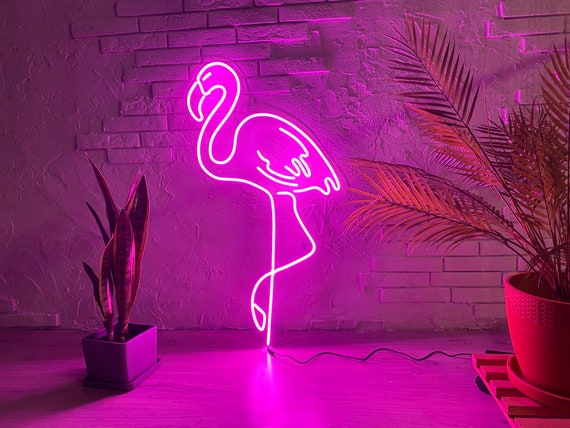The image showcases a room with a brick wall and a smooth concrete floor, both bathed in a purple glow from the vibrant lighting. Centrally placed in the scene is a neon sign in the shape of a flamingo with one leg raised and plugged into the wall for illumination. To the left of the neon flamingo is a potted plant with long, straight, and spider-like leaves that resemble a succulent. On the right side, a terracotta-style planter sits on a slotted wooden base, holding a lush fern with myriad leaves. The entire space is tinged with a pinkish-purple hue, creating a surreal and atmospheric ambiance that could suggest settings like a boutique, shop, or nightclub.